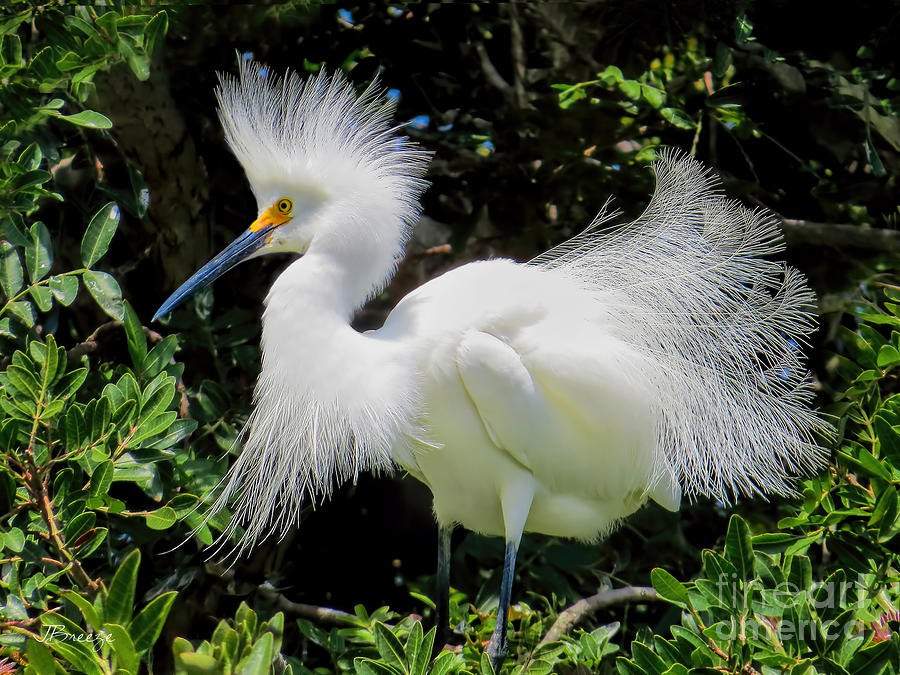This image features a magnificent white bird, possibly an egret, standing amid a lush green setting at the base of some trees. The photograph is taken up close, emphasizing the bird's striking features. The bird has a distinctive long black beak that transitions to an orangish-yellow hue near its sharp yellow eyes, which are outlined in orange with a black dot in the center. Its elegant neck forms an almost backward S shape, adding to its graceful appearance. Atop its head, a feathery crest or 'mohawk' delicately extends down its back, with each feather distinctly visible. The lower part of its neck boasts a loose, feathery beard. The bird's body is covered with soft white feathers that lie close to its skin, becoming more wispy and flowing towards the back and tail, giving an impression of lightness as if they could flutter with the slightest breeze. Although its long black legs aren’t fully visible in the photo, the detailed description highlights their presence. All around, the bird is framed by verdant plants and trees, further accentuating its pristine beauty.